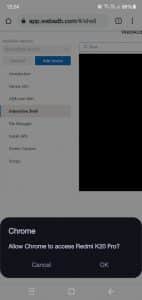This image depicts a web page viewed on a mobile device, but it is entirely blurry, making it difficult to discern specific details. The top part of the image appears to have text, but it is unreadable. There is a small settings icon visible, and a menu is displayed along the left-hand side. At the bottom of the screen, the text "chrome" and "chrome 2" is somewhat recognizable, accompanied by buttons labeled "Cancel" and "OK". A blue button is also present, but its text is illegible. The web page has a search bar, but its content cannot be deciphered. The image predominantly features shades of black, white, and gray, with the exception of the blue button. The blurriness obscures any information about the phone's status, such as the time or Wi-Fi connectivity, rendering the overall content of the web page incomprehensible.